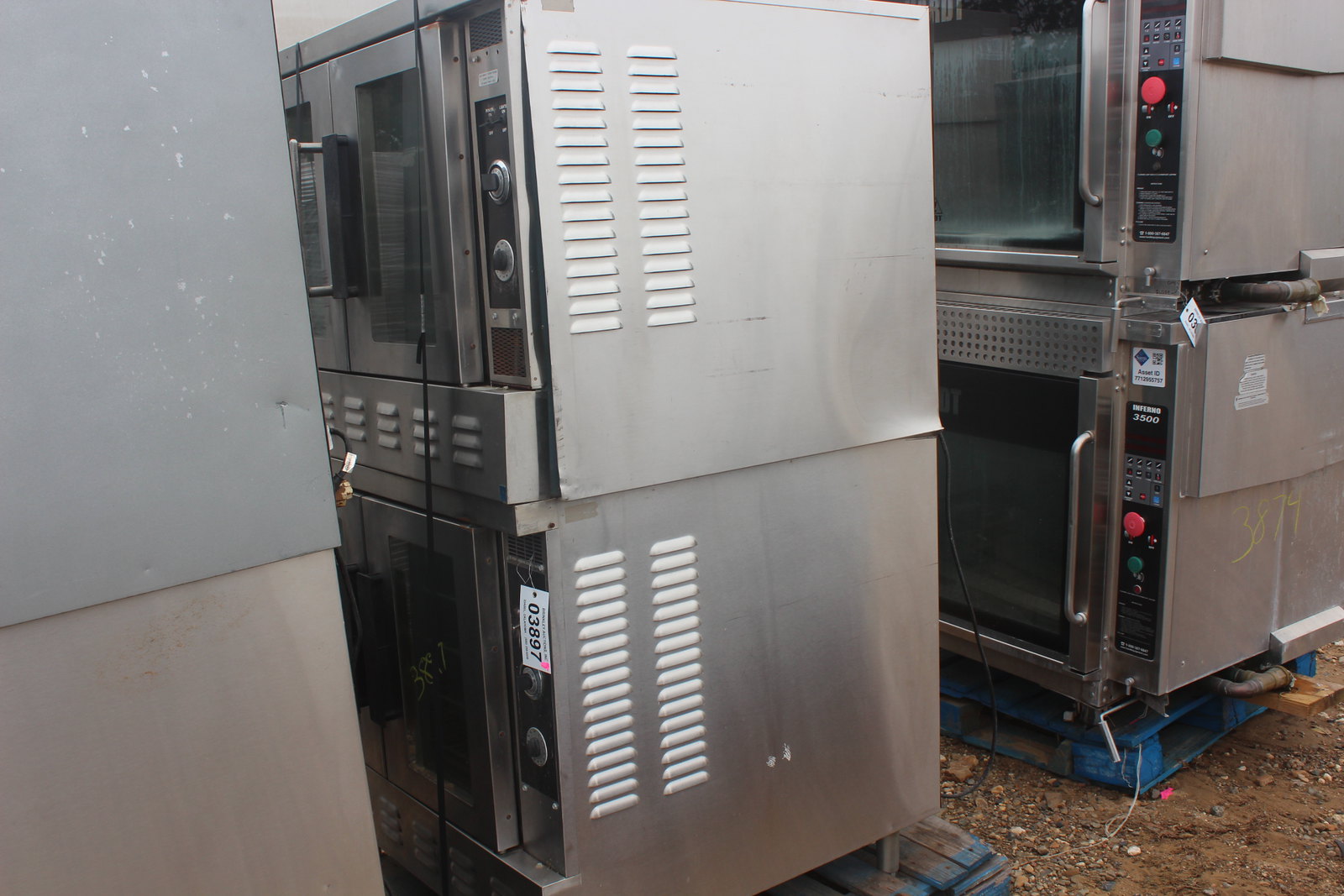This photograph features a set of large, industrial kitchen appliances, primarily ovens, that are situated outdoors. The appliances, constructed from various shades of stainless steel and silver, are arranged on blue-painted wooden pallets, placed on a ground of brown dirt and pebbles. The dirt and pebbles vary in color, including dark brown, light brown, white, and gray. 

There are four ovens in total, stacked in two pairs on each pallet. The pair on the left side has distinctive doors that open outward like French doors, equipped with dials on the side and glass fronts. The metal surfaces of these ovens show varying shades of gray, with the upper oven being a darker gray than the one below it. 

On the right side, the two ovens have larger doors with glass windows and are equipped with easily visible red and green buttons set within a black rectangle displaying white text. Immediately above the red button, a line of several pressable buttons is arranged. The control panels and vents are visible on the sides of these ovens, and each oven has a silver handle.

One of the appliances visible in the middle of the photograph has a tag with the number "03897" hanging from it, indicating it might be meant for inventory or identification purposes. The scene is well-lit, contributing to the outside ambiance of the photograph. This arrangement of appliances, likely waiting to be installed into a commercial kitchen environment, includes two distinct types of ovens characterized by different door mechanisms and control features.